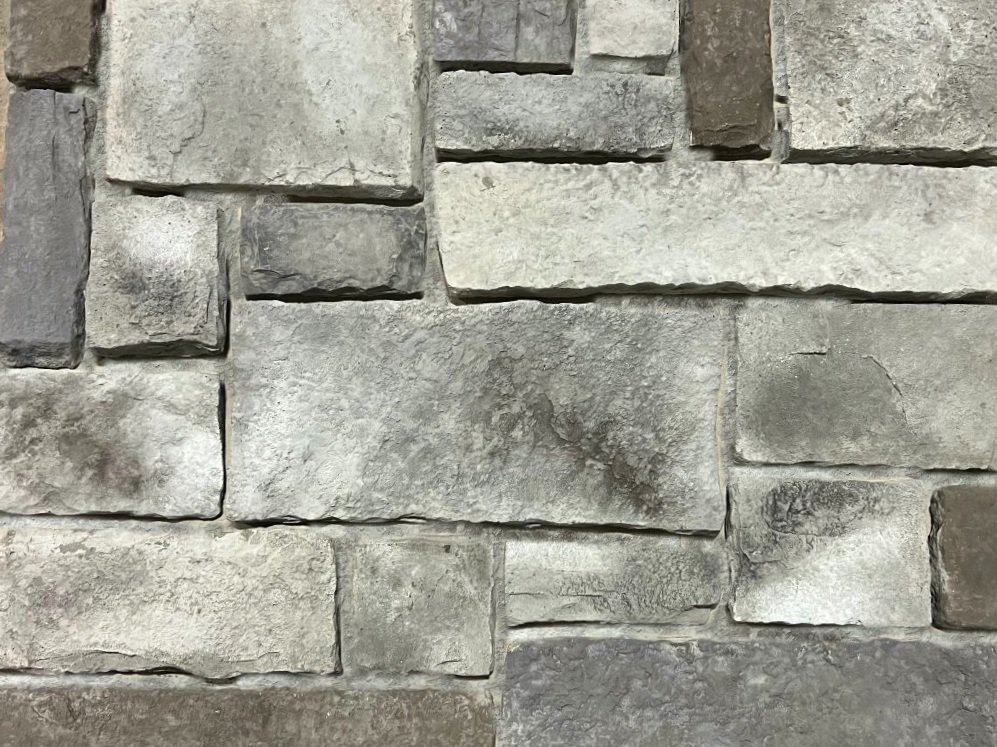This image showcases a close-up view of a stone masonry surface, which could either be part of a retaining wall or a walkway. The photograph captures an arrangement of flat stones of various shapes and sizes, predominantly rectangular and square. These stones are characterized by their irregular edges and are bound together with what appears to be concrete. The color palette ranges from light gray, very light white, and dark gray to shades of brown, giving a diverse and aged appearance. In the upper left corner, a large light gray square stone is prominent, below which and to the right, smaller rectangular and square stones continue the pattern. The overall composition of the stones, varying in color and size, creates an intriguing, textured mosaic effect.